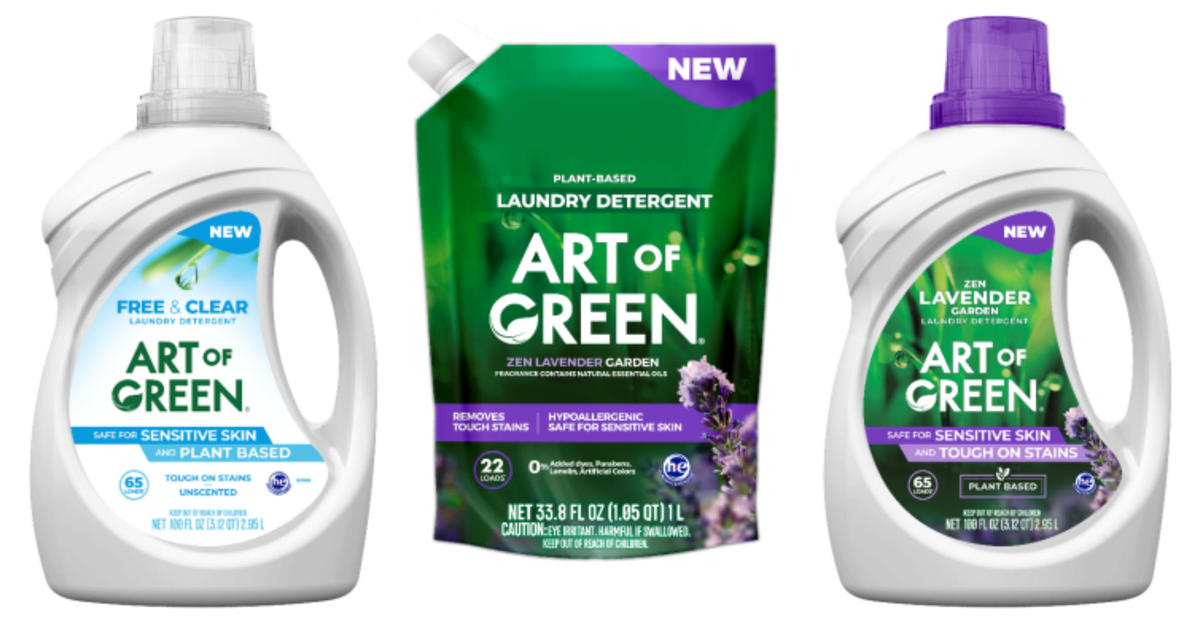This color photograph displays a trio of Art of Green laundry detergent products. Positioned on the left is a white plastic bottle with a clear cap, labeled "New Free and Clear Laundry Detergent." It highlights being unscented, plant-based, tough on stains, and safe for sensitive skin, accommodating up to 60 loads. Centrally, there is a green refill pouch with a pour spout, adorned with hints of purple, promoting "New Plant-Based Laundry Detergent" in the "Zen Lavender Garden" scent. This item, hypoallergenic and tough on stains, suits up to 22 loads. On the right, a gray bottle with a purple cap emphasizes the same "Zen Lavender Garden" scent, boasting similar features of being safe for sensitive skin, tough on stains, and plant-based, suitable for 65 loads. All products uniformly exhibit the "Art of Green" branding, catering to sensitive skin with eco-friendly, plant-based formulations.